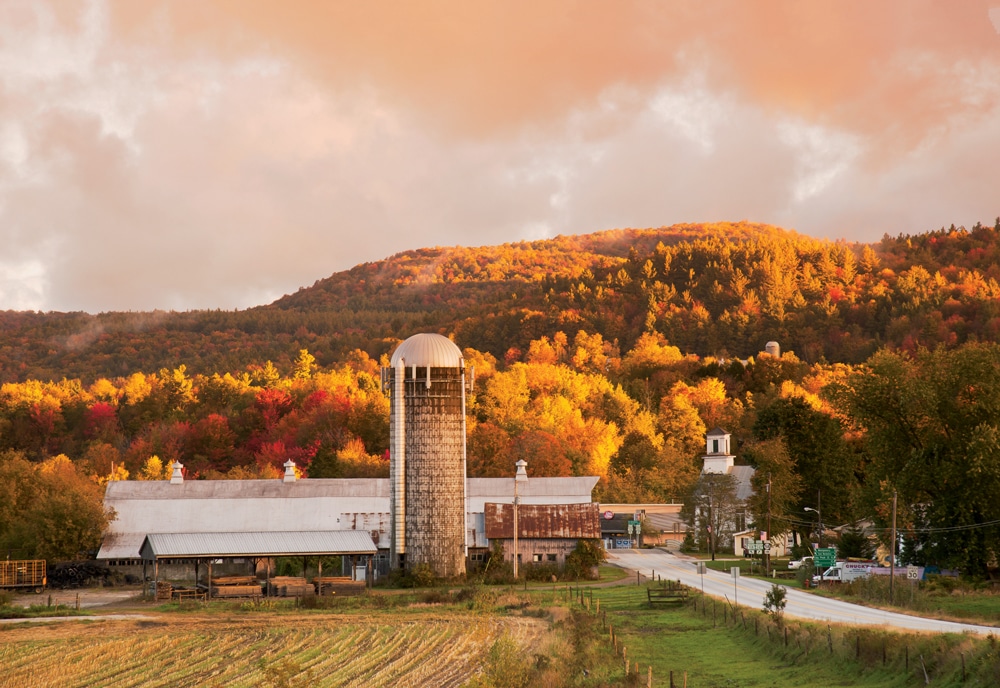Amidst a cloudy countryside scene, the photograph captures a large, weathered barn and a towering green silo, approximately 40 to 50 feet tall, set against a backdrop of a hilly landscape with vibrant fall foliage. The sky above is dark and gloomy with blueish-gray clouds and a hint of orange where the sun peeks through. In front of the barn and silo, freshly planted rows of crops stretch across the soil, bordered by patches of green grass. A smaller shed accompanies the larger structures. Further in the distance, a line of colorful trees in shades of yellow, red, and green define the horizon, with a mountain range visible above. Adjacent to the farm is a two-lane road, where a small city can be glimpsed, and several cars are parked nearby. The autumn leaves and harvest marks on the field complete this picturesque fall day on a bustling farm.